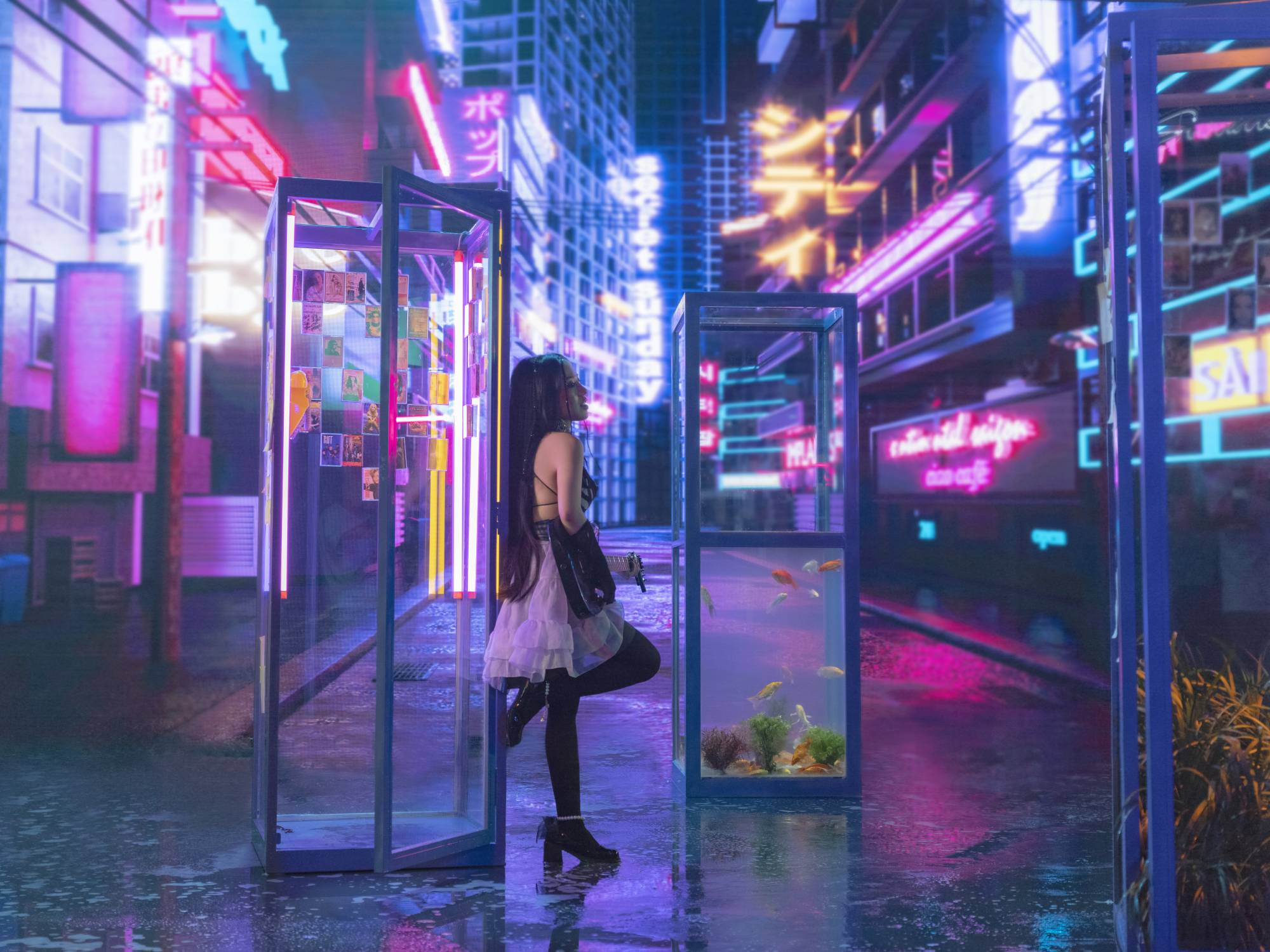In this night-time photograph of what seems to be a Japanese city, possibly Tokyo, vibrant neon lights and tall buildings encase a narrow, atmospheric alleyway. The ground is awash in the glow of florescent blues, pinks, mauves, and purples, casting an almost surreal luminescence over the scene. A striking young woman with very long, dark hair flowing almost to her buttocks, stands thoughtfully against one of three glass booths that line the alley. Her outfit consists of a frilly white skirt, a thin halter top, black leggings, and black booties adorned with bows. At the booth she leans on, the interior is decorated with Polaroid-type pictures, suggesting it might be a modern selfie booth. Another booth appears nearly aquatic, filled halfway like an aquarium, while the third booth teems with foliage. The night scene is blurry but alive with fluorescent colors and the mystery of urban life, punctuated by indecipherable white text on a building in the background.